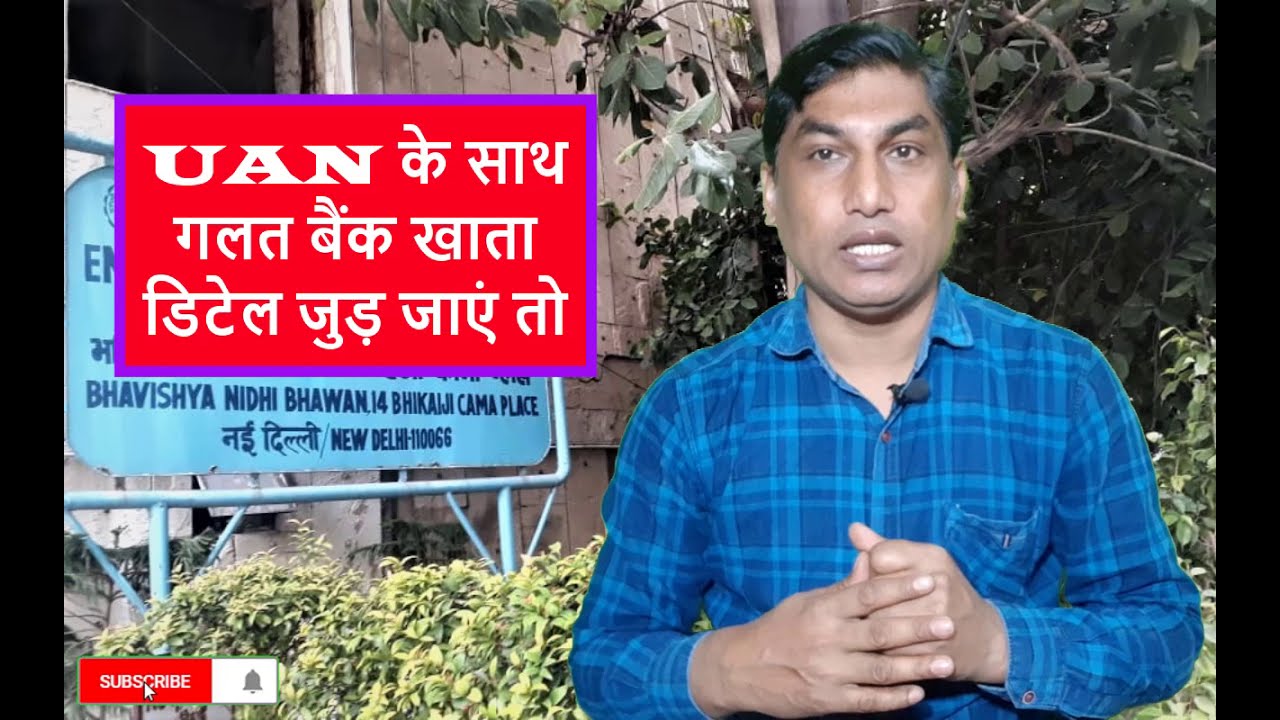The image captures a scene from a news media program, likely originating from India, possibly New Delhi. It features a Middle Eastern man positioned on the right side of the frame, with dark hair, eyebrows, and eyes. He is wearing a blue checkered shirt with a microphone clipped to his lapel, and his hands are clasped together in front of him. His mouth is open, revealing his lower teeth, suggesting he might be speaking.

He stands against a backdrop of green foliage and a building, with a tree trunk and abundant leaves visible behind him. To his left, there's a prominent metal sign displaying what appears to be location and direction information, partially obscured by a purple rectangle with a red border containing indecipherable white text. The red banner atop the sign also carries unreadable script.

In the bottom left corner, a red "Subscribe" button with a white bell icon indicates the likely presence of YouTube branding, suggesting this may be a social media or news channel screenshot. The entire image is bordered on the left and right by thin black lines, adding to the media-like presentation of the scene.